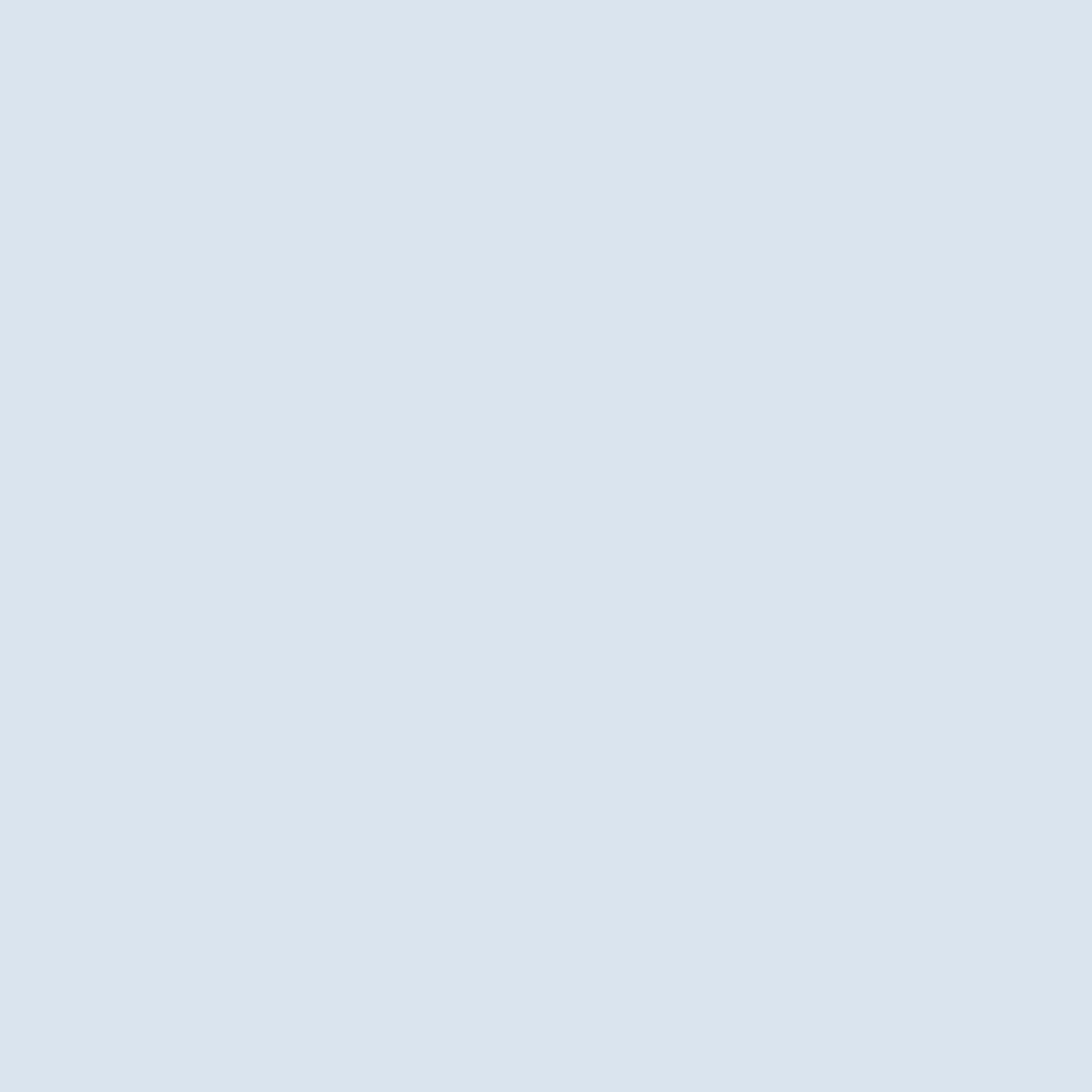The image depicts a blank square with a backdrop that exhibits a subtle bluish-gray hue. The color is best described as a pale gray with a hint of blue, reminiscent of a periwinkle shade but more subdued. There are no letters, shapes, or any other design elements present within the square. This minimalist and unadorned image potentially serves as a placeholder for an internet webpage or digital design project, offering a clean slate for further content or customization.